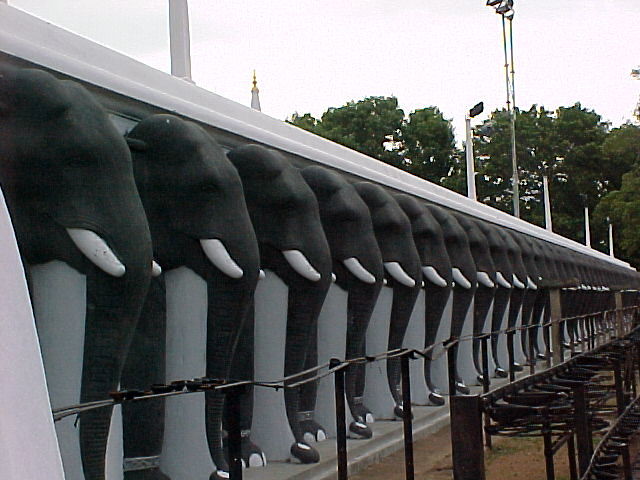In the image, there is a striking row of numerous elephant sculptures, standing side by side. These sculptures, numbering between 30 to 50, are rendered in a dark gray to black-green hue and feature short, white tusks. Notably, each sculpture has a slightly shining silver ring or bracelet around its ankles, possibly for identification. They appear to be situated within individual slots of a long, white partitioned structure reminiscent of horse stalls, with only their heads, trunks, and sometimes feet visible. The carefully crafted elephants lack eyes and mouths, emphasizing their artificial nature, possibly made from fabric or another material. In front of this arranged lineup, there is a metal pole fence, adding a structural element to the scene. The overall setting appears outdoor yet enclosed, creating a surreal and meticulous display.